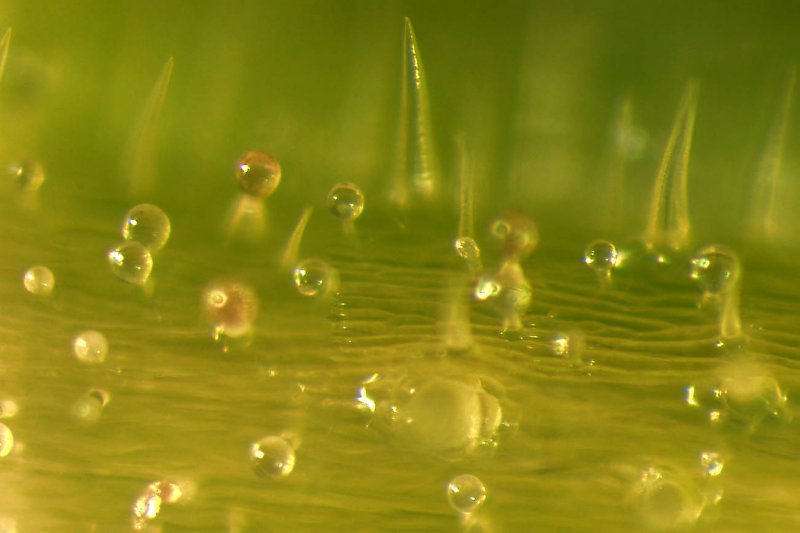The image depicts a murky scene dominated by a yellowish-green gradient that transitions from a more yellow hue at the bottom to a lighter green towards the top. The central focus is a larger body of water that appears contaminated, giving off an impression of pollution or a sewage environment. Water droplets and bubbles are visibly splashing and descending into this larger body of water, some of which have a reddish-brown tint, adding to the sense of contamination. The surface of the water is dotted with translucent, circular droplets resembling bubbles, adding texture and visual interest. In the blurred background, there are elongated, translucent shapes that resemble thick blades of grass with pointy tops, contributing to the overall eerie and mysterious atmosphere of the image. The scene exudes an impression of a polluted, almost otherworldly liquid environment with a greenish-yellow glow and numerous spiky and spherical water droplets.